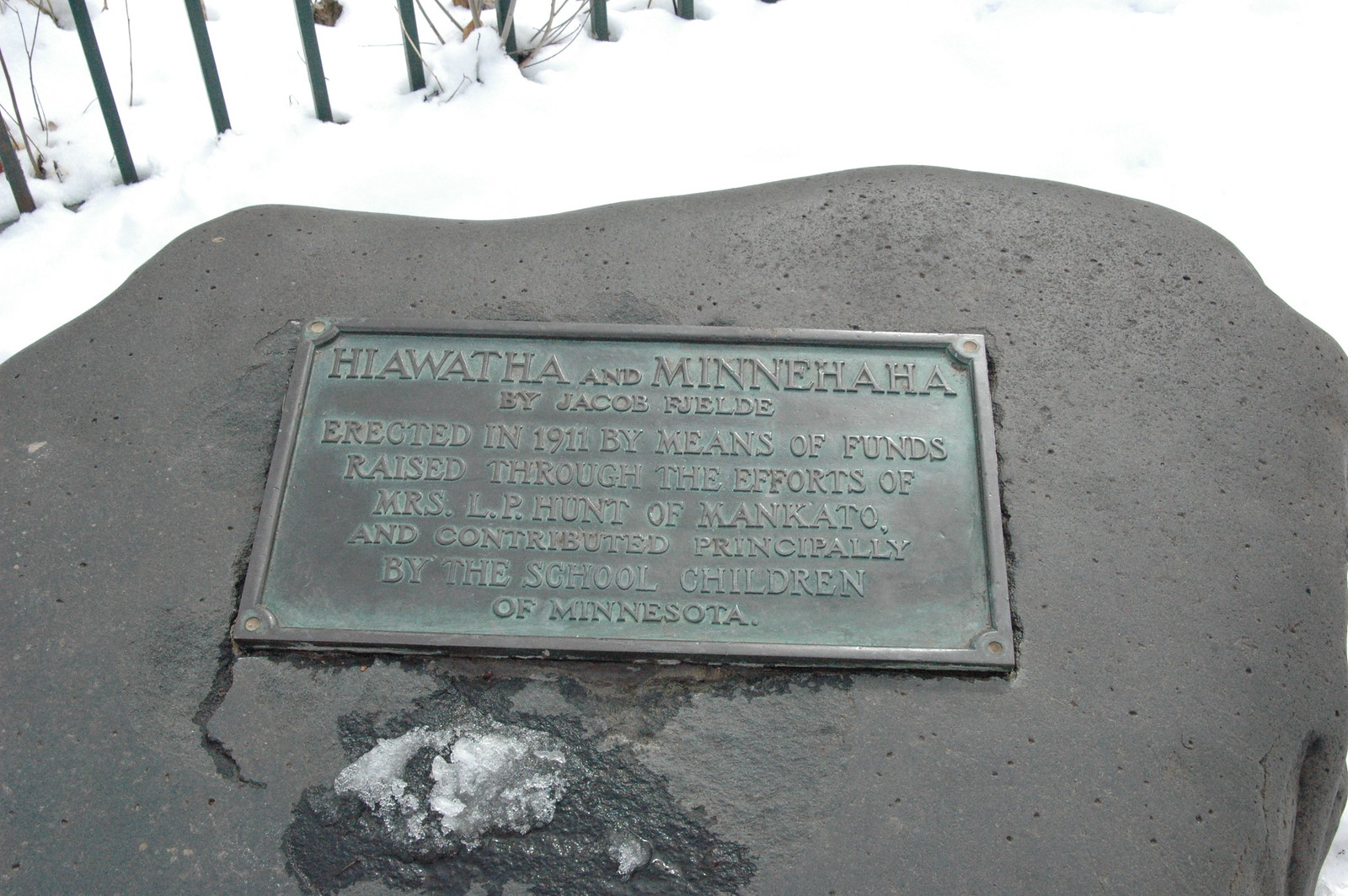This image depicts a large, smooth, gray stone with a brass plaque displaying a greenish patina, indicating age. The plaque, set in the stone like a plate, is dedicated to "Hiawatha and Minnehaha by Jacob Fields." It was erected in 1911 through funds raised by Mrs. L. P. Hunt of Mankato, principally contributed by the schoolchildren of Minnesota. The scene is set in a wintry landscape, with snow covering the ground and a black metal fence visible behind the stone. Some sticks or plant stems poke through the snow, and there is even some ice visible on the stone in the foreground, adding to the overall cold, serene atmosphere.